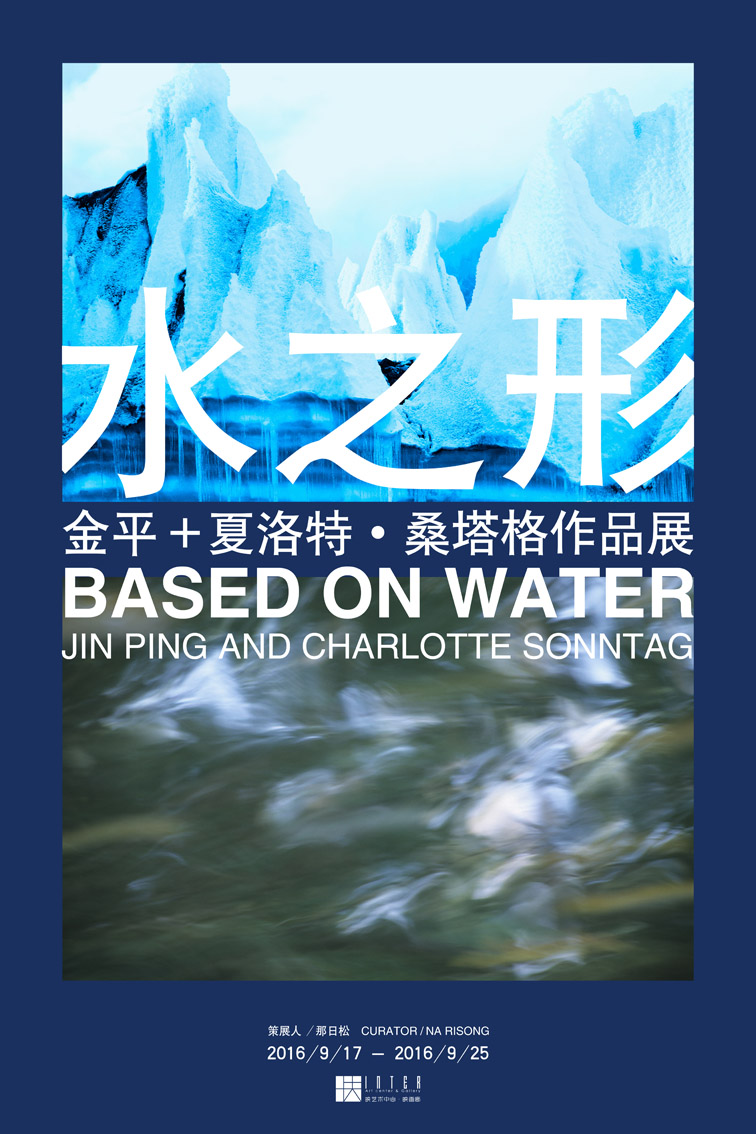The image appears to be a vertically-oriented poster with a dark navy blue border. At the center are two stacked rectangular photographs. The top photo showcases jagged, icy mountains or glaciers with a striking light blue hue. Overlaid on this top image are three large white Chinese characters. Below this, a wide navy blue stripe, matching the border, contains additional Chinese characters. 

Directly beneath the stripe is a second photograph depicting rippling water, possibly a stream or pond, with visible white reflections and potentially blurred fish beneath the surface. Superimposed on this water image is the text "Based on Water" in a larger white font, followed by the names "Jin Ping and Charlotte Sontag" in a smaller white font.

Set against the dark blue background between the two photographs is a cluster of Chinese characters. Furthermore, at the bottom of the image, centered on the dark blue border, more Chinese characters are written in white, alongside the text "Curator: N.A. Rysong." Below this, it states the dates "2016/9/17 - 2016/9/25," followed by an indistinguishable logo.